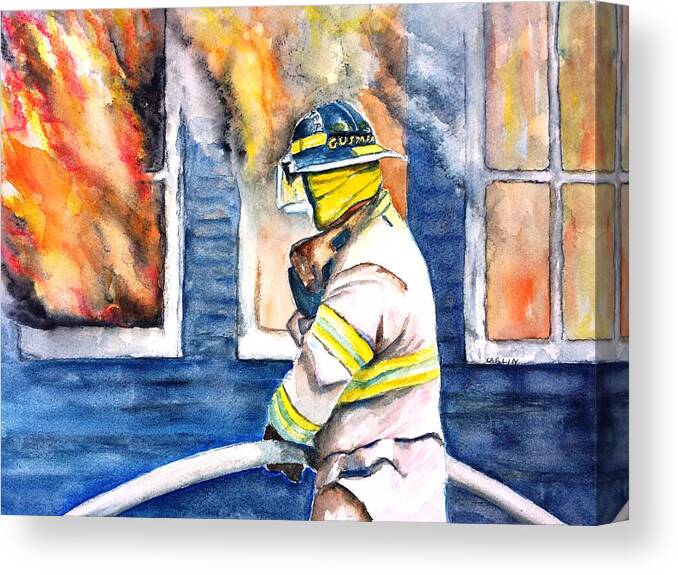This artwork, presented in a cartoonish watercolor style, portrays a dramatic scene where a firefighter is battling an intense blaze outside a blue wooden home. The firefighter, centered prominently in the composition, is dressed in a white jacket with distinctive yellow stripes. His face is completely covered by a yellow cloth and he wears a plastic face shield, while a blue helmet with the name "Guzman" on a dark blue label rests on his head. A respirator hangs around his neck. He grips a white hose firmly with his black-gloved hands as it droops toward the ground.

Surrounding the firefighter, the house is engulfed in vivid red and yellow flames, with thick black smoke pouring from the windows. There are three windows depicted: the far left window is shattered with aggressive flames and smoke billowing out; the center window is likewise broken, showing a mix of flames and smoke; and the rightmost window, yet to be broken, reveals fire and smoke struggling to escape through the intact pane. This intense, chaotic scene highlights the peril and bravery of the firefighter in the face of overwhelming danger.